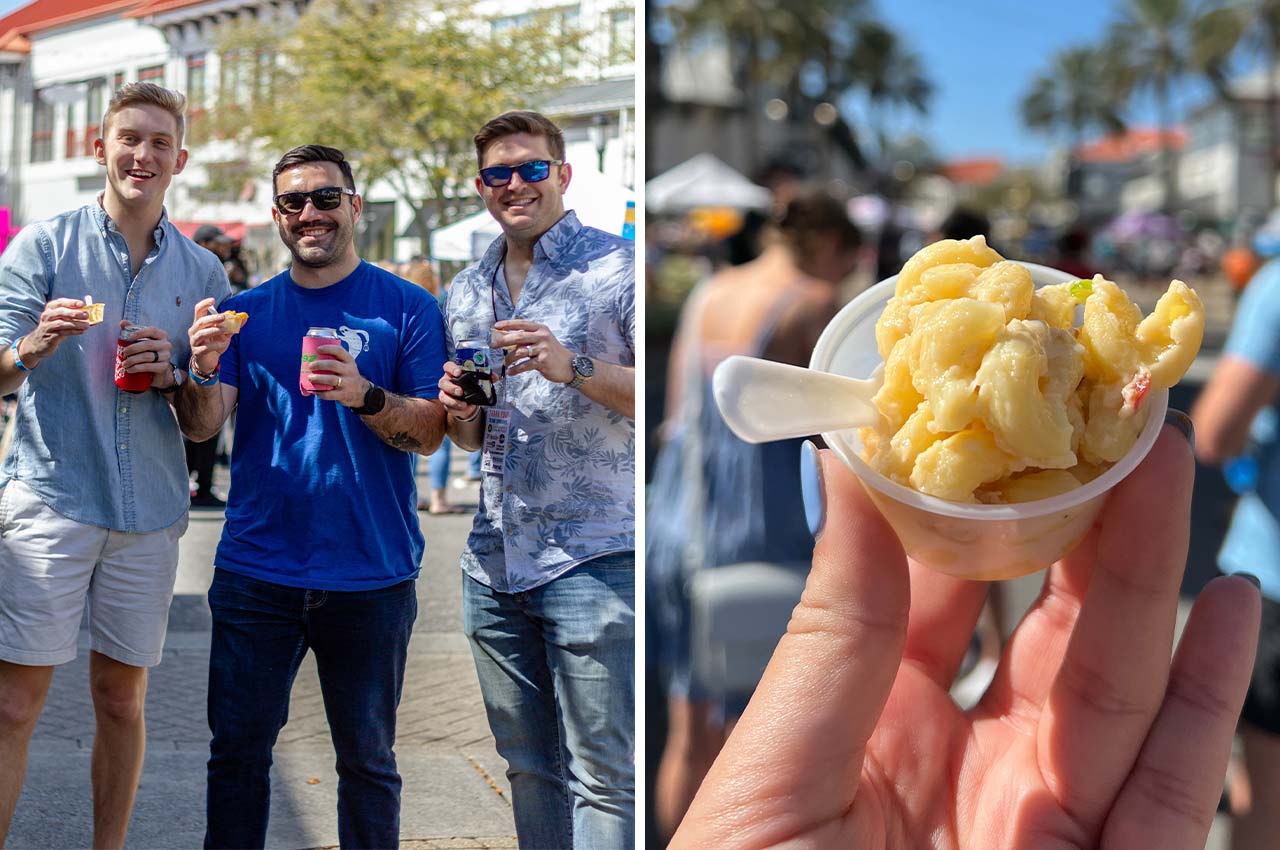Two side-by-side photographs depict a vibrant outdoor food and beverage festival. The image on the left showcases three young Caucasian men of varying heights, two of whom wear sunglasses, each holding up small plastic ramekins filled with mac and cheese in one hand and beverage cans in cooler cozies in the other. The third man has reversed the hands holding the items. Against a backdrop of clear blue skies and palm trees, with crowds of people adding a bustling atmosphere, this scene captures a warm, sunny day. The image on the right offers a close-up of the macaroni and cheese, framed by a woman’s hand adorned with lavender nail polish, further emphasizing the cozy festival ambiance on a busy city street.